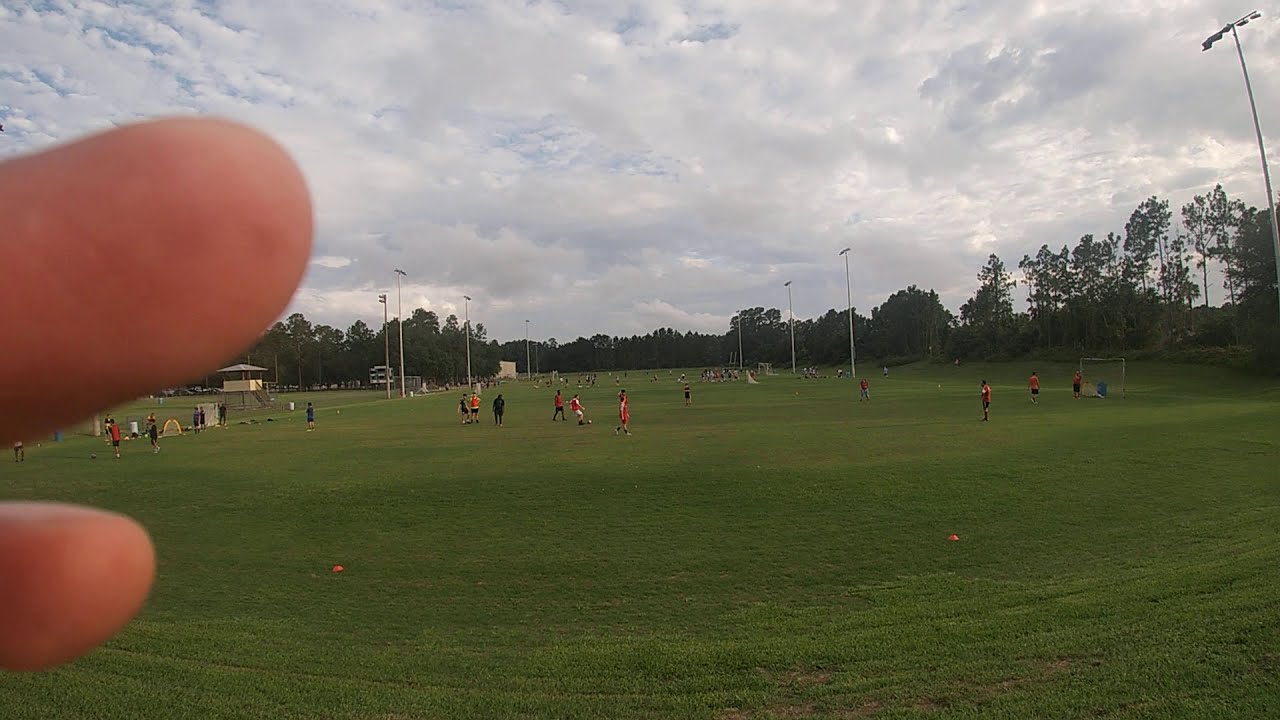The image captures a lively soccer match on a meticulously maintained, short green grass field, under a dramatic sky filled with dark gray clouds. Multiple players are dynamically engaged in the game, wearing red and black uniforms, and focusing on a white soccer ball positioned in the center. The soccer field is framed by various green-leaved trees that add a natural border. On the right side, a black net with white poles stands ready to receive any incoming goals, while orange cones clearly mark the play area's boundaries. However, the left side of the image is partially obscured by the photographer's two fingers. In the distance, tall poles, possibly for nighttime game lights, can be seen, hinting at the versatility and extended use of the field. The combination of these elements evokes a sense of anticipation, as the dark gray clouds suggest an impending storm.